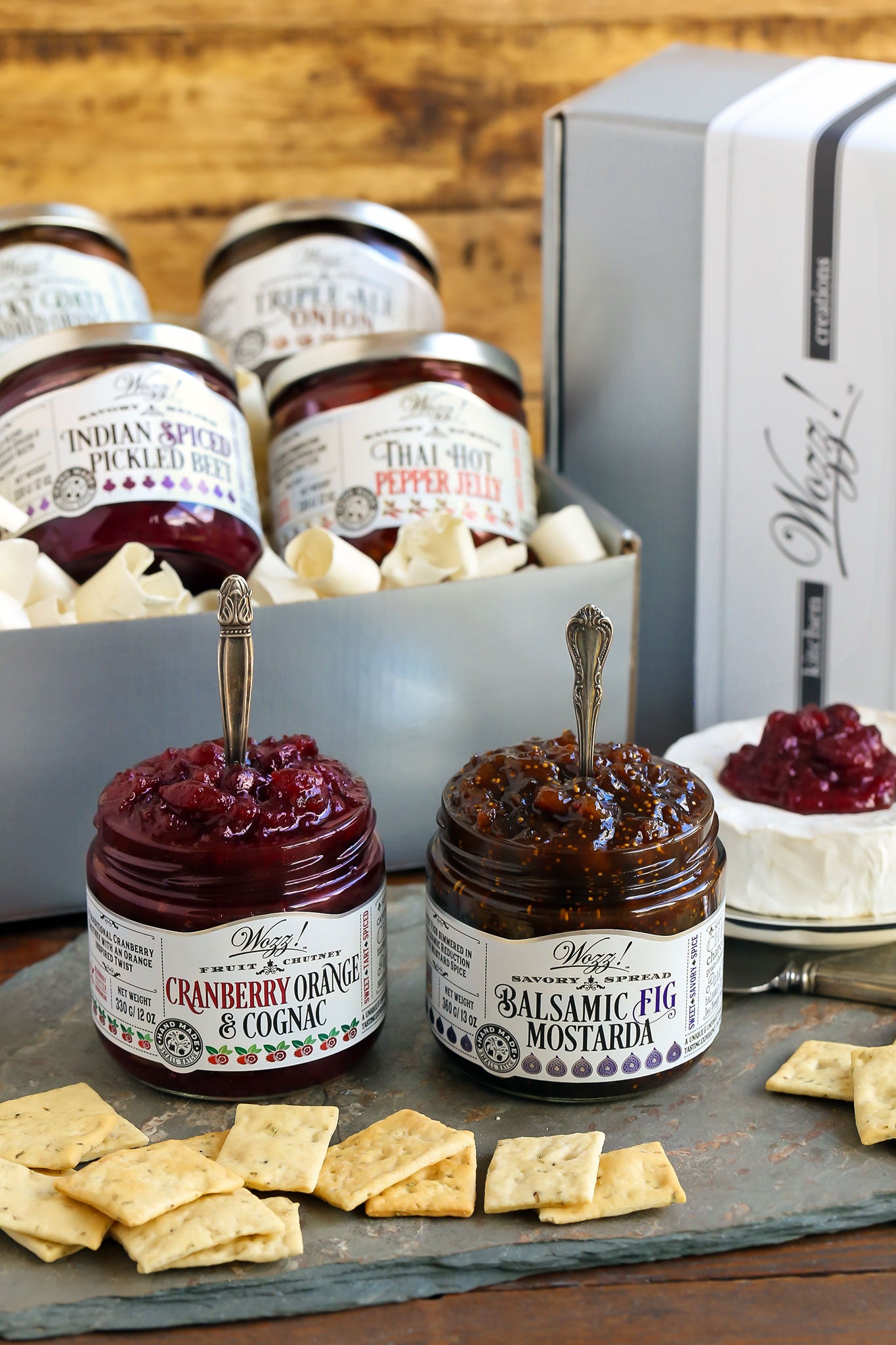The image showcases a sophisticated cheese board arrangement set on a piece of slate atop a wooden table. Central to the display is a wheel of brie, adorned with a dollop of jam, and accompanied by a cheese knife. The setup highlights two open jars of jam: "Cranberry Orange and Cognac" with a deep red hue and "Balsamic Fig Mostarda" exhibiting a dark reddish-brown color. Both jars, cylindrical and short with white labels, have small spoons or knives sticking straight up from them. Scattered around the cheese board are tan square crackers, adding texture and crunch to the presentation. In the background, a box containing four additional jars of various spreads labeled "Triple Ale Onion," "Indian Spice Pickle Beet," "Thai Hot Pepper Jelly," and other intriguing flavors can be seen, providing a sense of variety and culinary exploration.